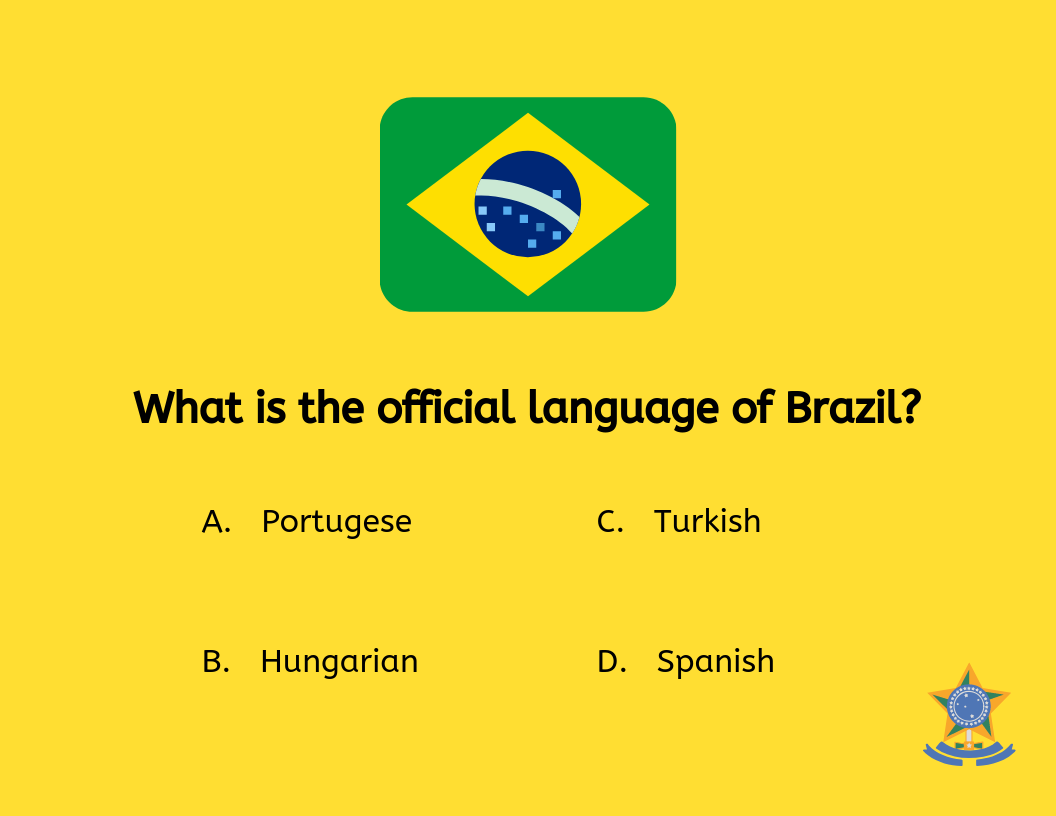The image features a bright yellow background, resembling a trivia question layout. At the top center, a Brazilian flag is prominently displayed. The flag consists of a green rectangle with a yellow diamond in the center, inside which there is a blue globe adorned with stars.

Beneath the flag, the question "What is the official language of Brazil?" is written in bold, non-serif font. Below the question are four answer options arranged in two columns:

- Top left: A. Portuguese
- Bottom left: B. Hungarian 
- Top right: C. Turkish
- Bottom right: D. Spanish

In the bottom right corner of the image, there is a logo consisting of a five-pointed star with a blue circle inside. Below the circle, there are two blank blue ribbons without any text.

The overall design of the image is quite simple and plain, suggesting that it might be used in a learning app or similar platform for trivia questions.